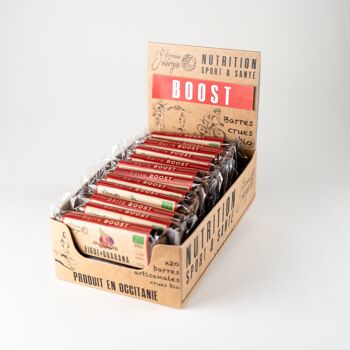The photograph showcases the energy bar product “Boost,” presented in a staged setup against a white backdrop. The product is contained within a beige, rectangular cardboard display case that holds several smaller packages. The focal point is a striking red banner with the brand name "Boost" in bold, white letters, prominently displayed in the center of the box. The packaging includes various elements that indicate its nutritional purpose and sports-oriented use, with phrases like "Nutrition" and "Sport" visible. The box also features illustrations of people on bicycles, suggesting its appeal for athletes, potentially cyclists like those in the Tour de France, needing an energy boost for endurance. Language cues, including terms like “Product in Occitane” and other French phrases, indicate that the product is likely from a French-speaking region. Each individual bar within the box has distinct features such as a greenish square in the corner and a purplish image, further defining the product's branding.